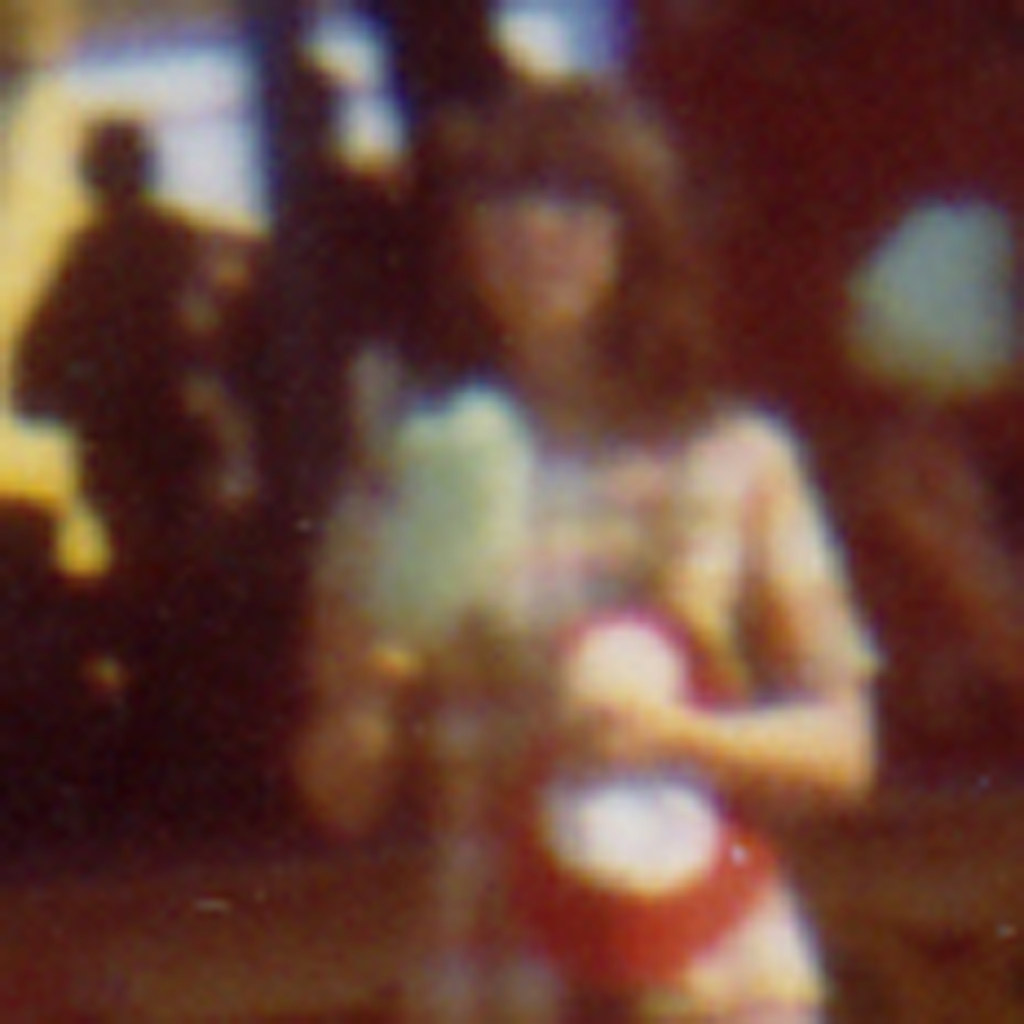The photograph is an extremely blurry image of a woman with shoulder-length brown hair styled with straight bangs across her forehead. She appears to be facing the camera and wearing a short-sleeved top that has a plaid pattern incorporating colors like tan, red, yellow, white, and pink. The lighting in the photograph is very poor, rendering her facial features indistinguishable.

In her right arm, she holds what looks like a red and white object, potentially a stuffed animal. Her left hand is raised and seems to be holding something green and possibly puffy, likely cotton candy. The background is dark and poorly lit, though faint details reveal the silhouettes of at least two people on the left side, surrounded by a mix of faded red, yellow, and blue hues.